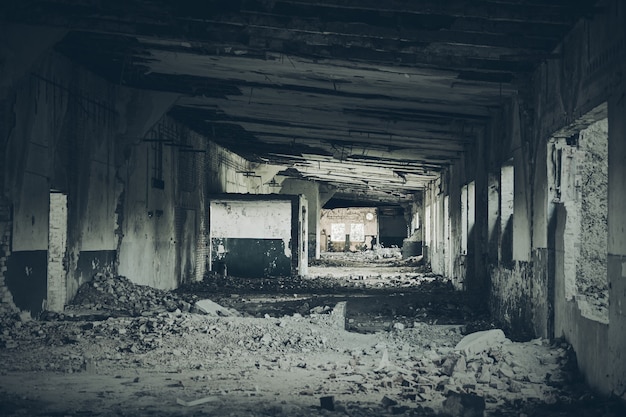The image depicts a dimly lit, grayscale interior of an old, decrepit building, possibly situated under a bridge or tunnel-like structure. The scene is dominated by an abundance of crumbling concrete blocks, dust, and debris strewn across the floor, indicating long-term abandonment. The right-hand wall is lined with window openings that lack any glass, allowing patches of light to filter into the otherwise dark space. The ceiling, distinguished by its slight angle descending from left to right, contributes to the shadowy atmosphere in the foreground, with a subtle increase in illumination further back. The left side features a primarily concrete wall adorned with a darker band along the bottom third, along with a couple of open doorways leading deeper into the corridor. Metal poles protrude from the walls, and scattered detritus, particularly around the windows and doorways, add to the sense of neglect and decay. The pervasive gray hues and a slight greenish tint further emphasize the building's forlorn and forgotten state.